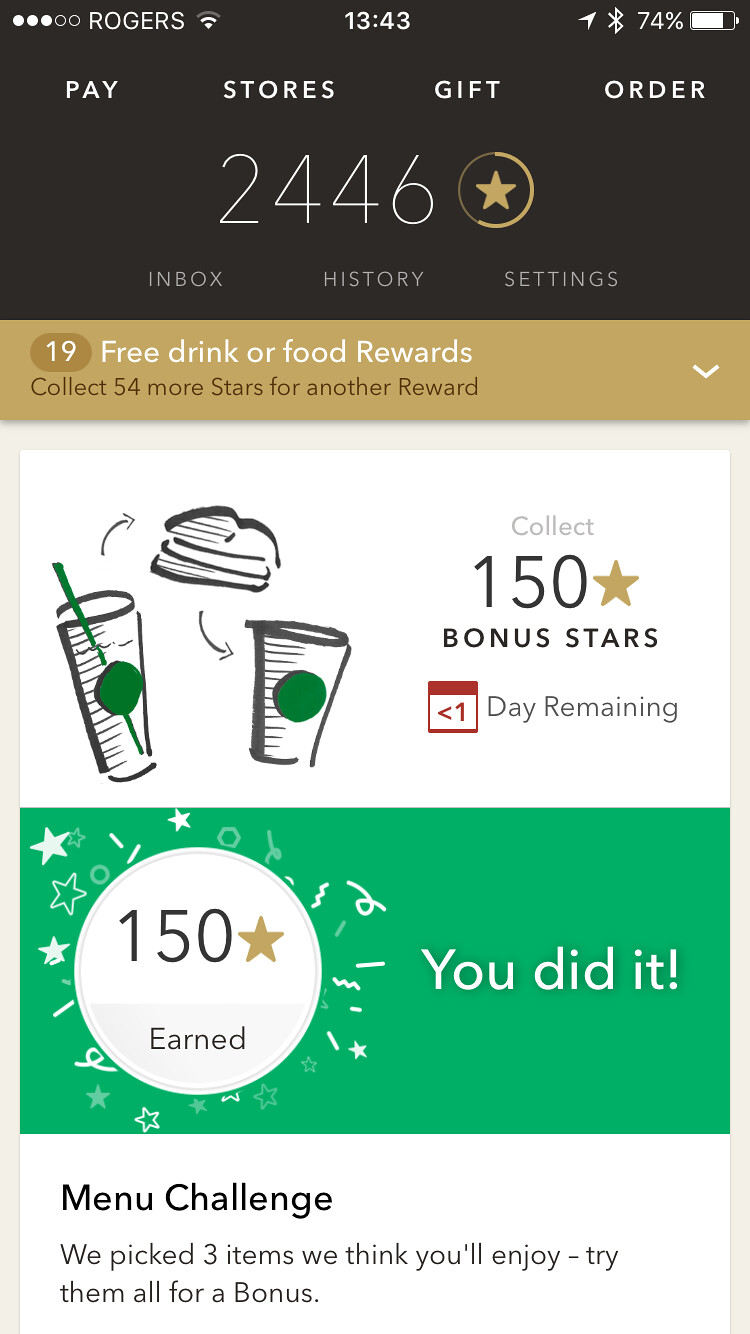The image is a screenshot from the Starbucks app on a cell phone. At the top of the screen, there are four tabs labeled "Pay," "Stores," "Gifts," and "Orders." Below that, it displays "2446" with a star icon next to it, indicating the user's points or stars. Further down, there are options: "Inbox," "History," and "Settings." The screen also shows a gold bar highlighting "19 free drink or food rewards," and it mentions that collecting 54 more stars will earn another reward. Beneath this, a notice in a white section prompts, "Collect 150 bonus stars in less than one day remaining." The section is visually divided, with two cartoonish Starbucks drinks and a sandwich illustrated alongside a green circle featuring celebratory icons such as stars and confetti, saying "You did it." Additionally, it displays a "Menu Challenge," explaining, "We picked three items we think you'll enjoy. Try them all for a bonus," though it doesn’t specify the items. The phone is on the Rogers network with three out of five bars of Wi-Fi signal, the current time is 13:43, and the battery is at 74%.